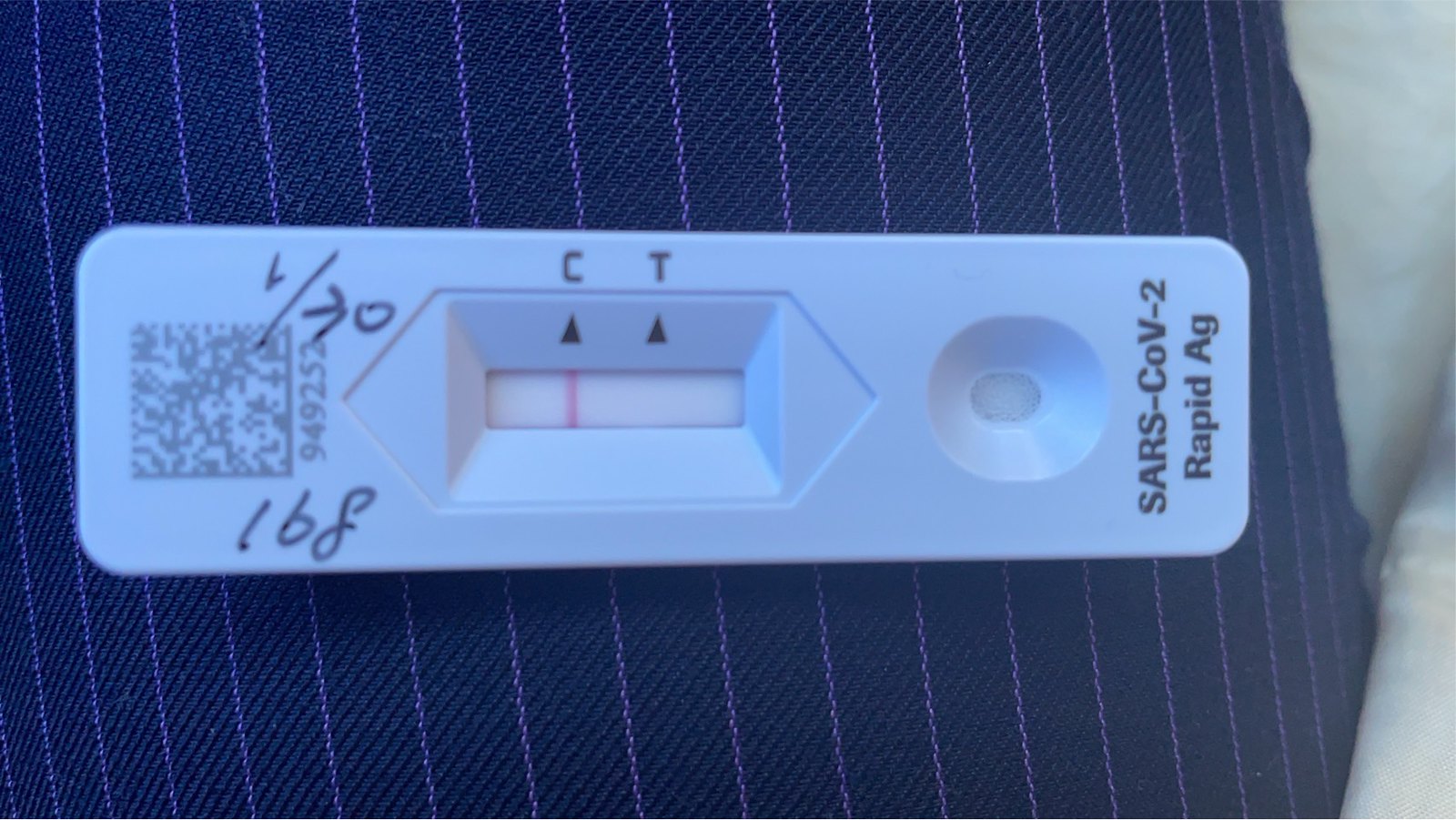This underexposed, low-contrast photograph depicts a SARS-CoV-2 rapid antigen test device. Positioned horizontally in landscape mode, the white plastic test device occupies most of the image's width and about a third of its height. It rests on a dark blue cloth featuring subtle purple single-stitch stripes. To the right, there's an indistinct, puffy white object, possibly another piece of fabric.

The test device itself is marked with several notable features. On its left side, a two-dimensional barcode is visible with the number "949252" printed below it. Some upside-down text can be seen, potentially reading "168" or "86, 891" depending on its orientation. There's also some ambiguous writing that includes a fraction (one slash) and a pointer to zero. The right side of the device is labeled clearly with “SARS-CoV-2 Rapid AG,” indicating its function as a rapid antigen test for COVID-19.